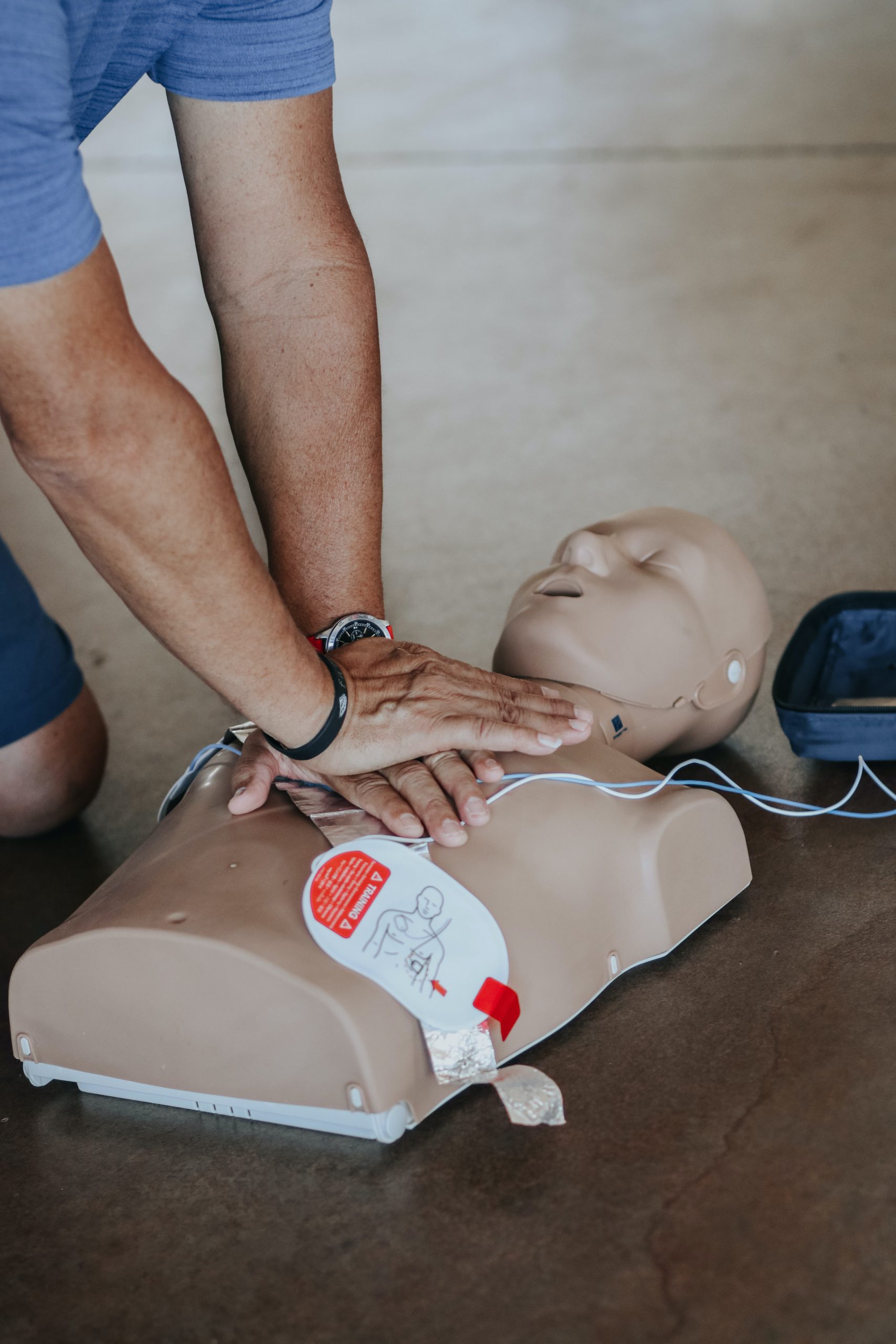In this detailed image, a man is performing CPR on a beige-colored plastic dummy which is placed on the ground. He is dressed in a dark blue t-shirt and matching blue shorts, his arms are bare, revealing a scuba diving watch on his left wrist. His hands are positioned correctly with his right palm over his left, executing chest compressions on the dummy. The scene captures his effort to sustain a heartbeat by applying rhythmic pressure. Attached to the dummy's chest are white and blue wires leading to a small machine, indicative of medical monitoring or training equipment. Additionally, a white label with red detailing is affixed to the dummy, providing instructions for the CPR procedure. There is no text overlaid on the photo, allowing clear focus on the life-saving practice.